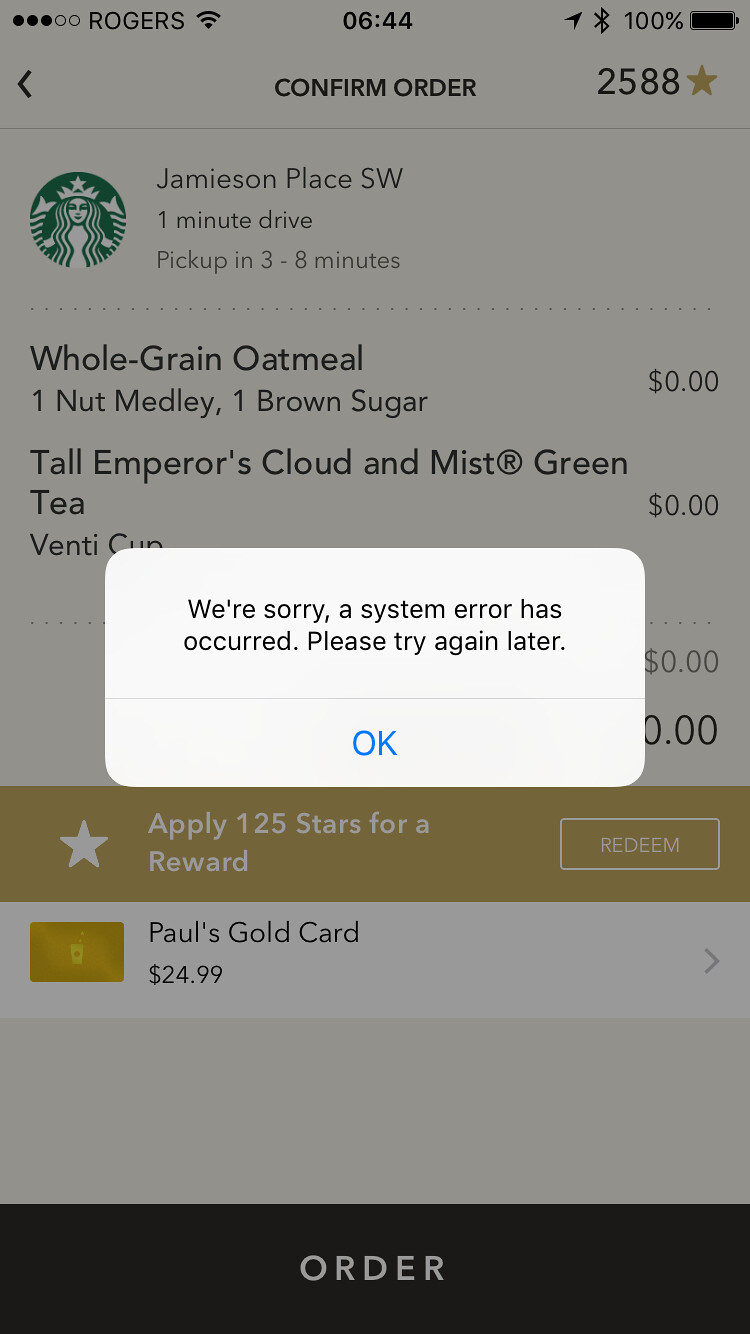A screenshot of a phone displaying a Starbucks order. Centered is a white popup box with a curved edge, containing black text that reads, "We're sorry, a system error has occurred. Please try again later." Beneath the message is a thin line and a yellow "OK" button.

At the top of the phone screen, the status bar indicates various elements: the signal strength icon shows five dots (three black, two white), the carrier "Rogers," a Wi-Fi icon, the time "06:44," an arrow pointing up to the right, a Bluetooth symbol, "100%," and a battery icon. Beneath the status bar, the first line of text features a left-pointing arrow, "Confirm Order" in the center, and "2588 ★" on the right.

Next, a line displays the Starbucks logo on the left, accompanied by the address "Jameson Place SW," a note that it's "One minute drive," and “Pick up in three to eight minutes.” The order details follow, listing "Whole Grain Oatmeal" with "One Nut Medley" and "One Brown Sugar," marked at zero dollars. Below it, "Tall Emperor's Cloud and Mist Green Tea" is shown with zero dollars on the right, and partially obscured text below indicates a "Venti Cup."

Further down, a brown bar with a white star and "Apply 125 stars for a reward" next to a redeem button is present. Below this section is an image of a gold card labeled "Paul's Gold Card," showing a balance of 2499 stars. At the bottom of the screen, a black bar with white text reads "Order," indicating the button for placing the order.

Overall, the screenshot captures a failed attempt to place a Starbucks order, overlaid by an error message that halted the transaction.